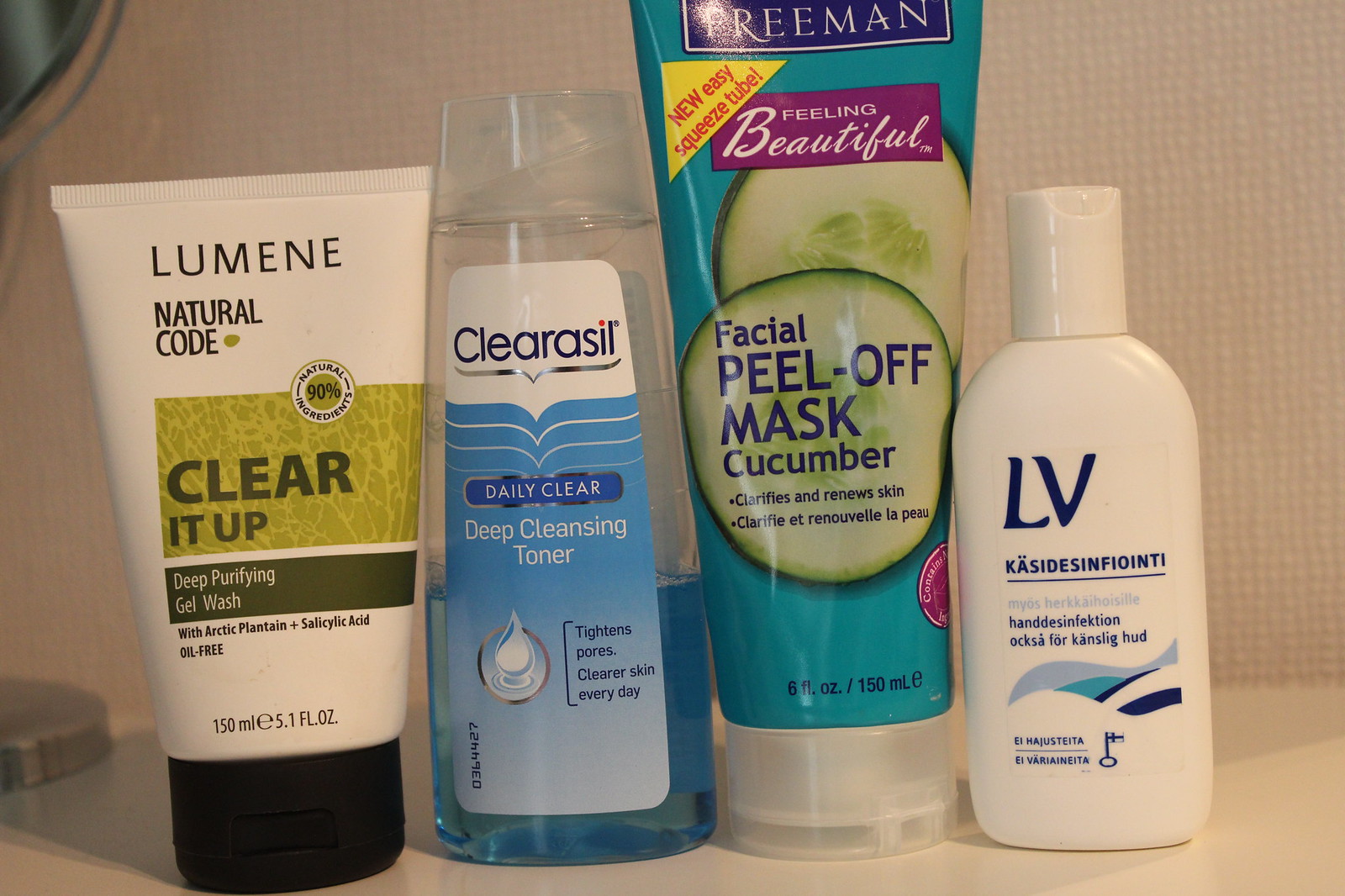The photograph features a beige wall in the background with a white surface in the foreground. On the left side of the white surface, there is a metallic round object. Additionally, the surface is occupied by four plastic bottles arranged from left to right. 

The first bottle on the left is white with a black cap facing downwards and a green label. It is labeled "Lumine Natural Code Cleared Up Deep Purifying Gel Wash with Arctic Plantain and Salicylic Acid, Oil-Free, 150 milligrams, 5.1 fluid ounces." 

Next to it is a clear plastic bottle about halfway filled with a blue liquid. It has a white and blue label that reads "Clearasil Daily Clear Deep Cleansing Toner Tighten Pores, Clear Skin Every Day."

To the right of that is a bottle with a clear white cap at the bottom and a label in turquoise, yellow, and purple. The label states "Freeman New Easy Squeeze Feeling Beautiful Facial Peel-Off Mask, Cucumber, Clarifies and Renews Skin, 8 fluid ounces, 150 milliliters."

The last bottle on the far right is a white plastic bottle with some text in Swedish and the label "LV" at the top.